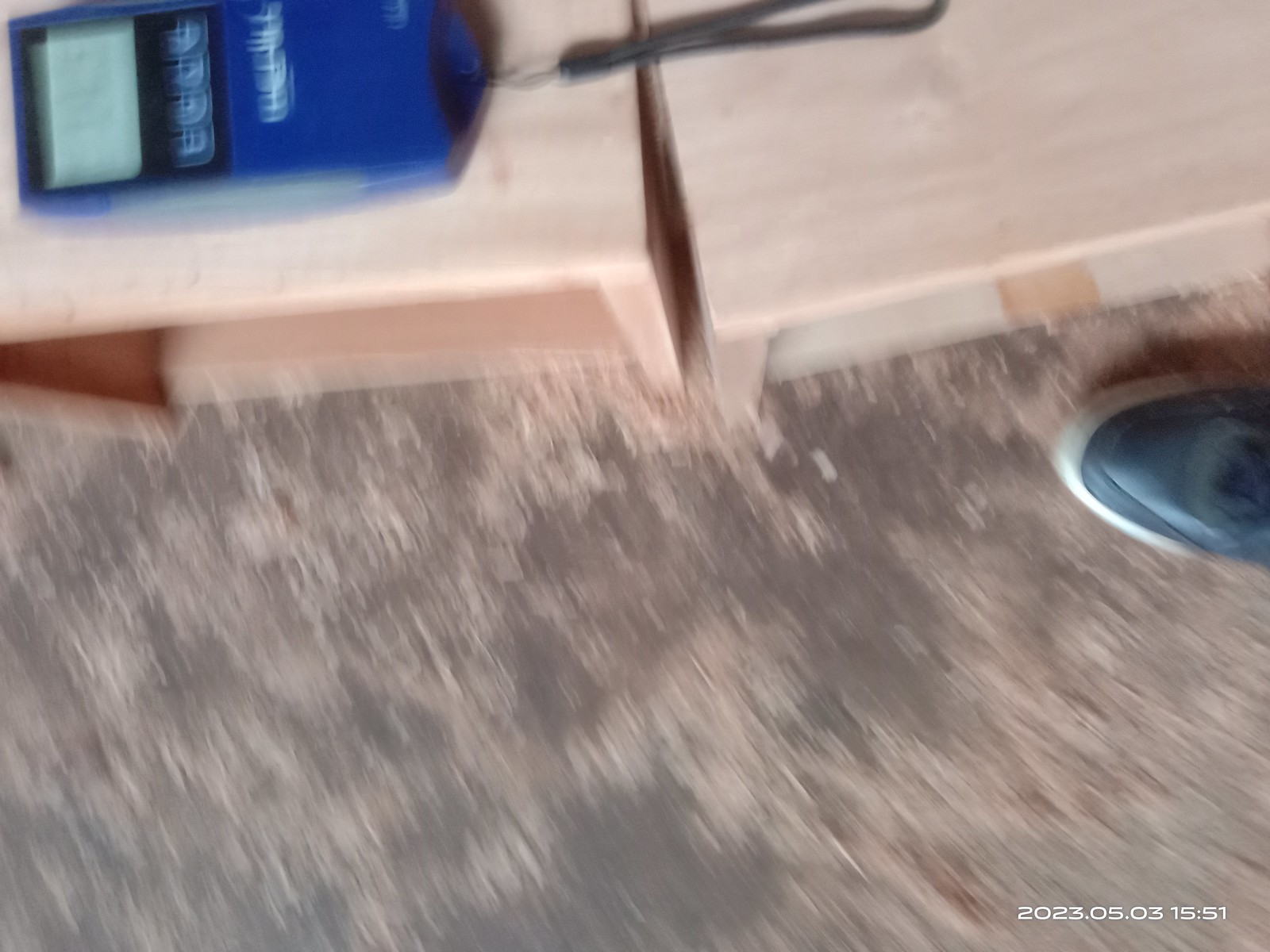In this realistic yet blurry photograph, likely captured while the person was in motion, the scene depicts two distinctive wooden tables or stands. The shorter stand on the right has a simplistic flat design with limited space for storage. In contrast, the taller stand on the left features two legs on either side and an open middle section ideal for placing items. The discolored floor beneath, marked by gray and tan splotches, appears to have faded paint. A black shoe with black laces and white trim is partially visible in the bottom right corner of the image. Positioned atop the left stand is a blue electronic device, which has a screen and four buttons beneath it, with a black keychain dangling from its base. The date "5-3-15-15" is marked at the bottom, despite the picture being taken in 2023.